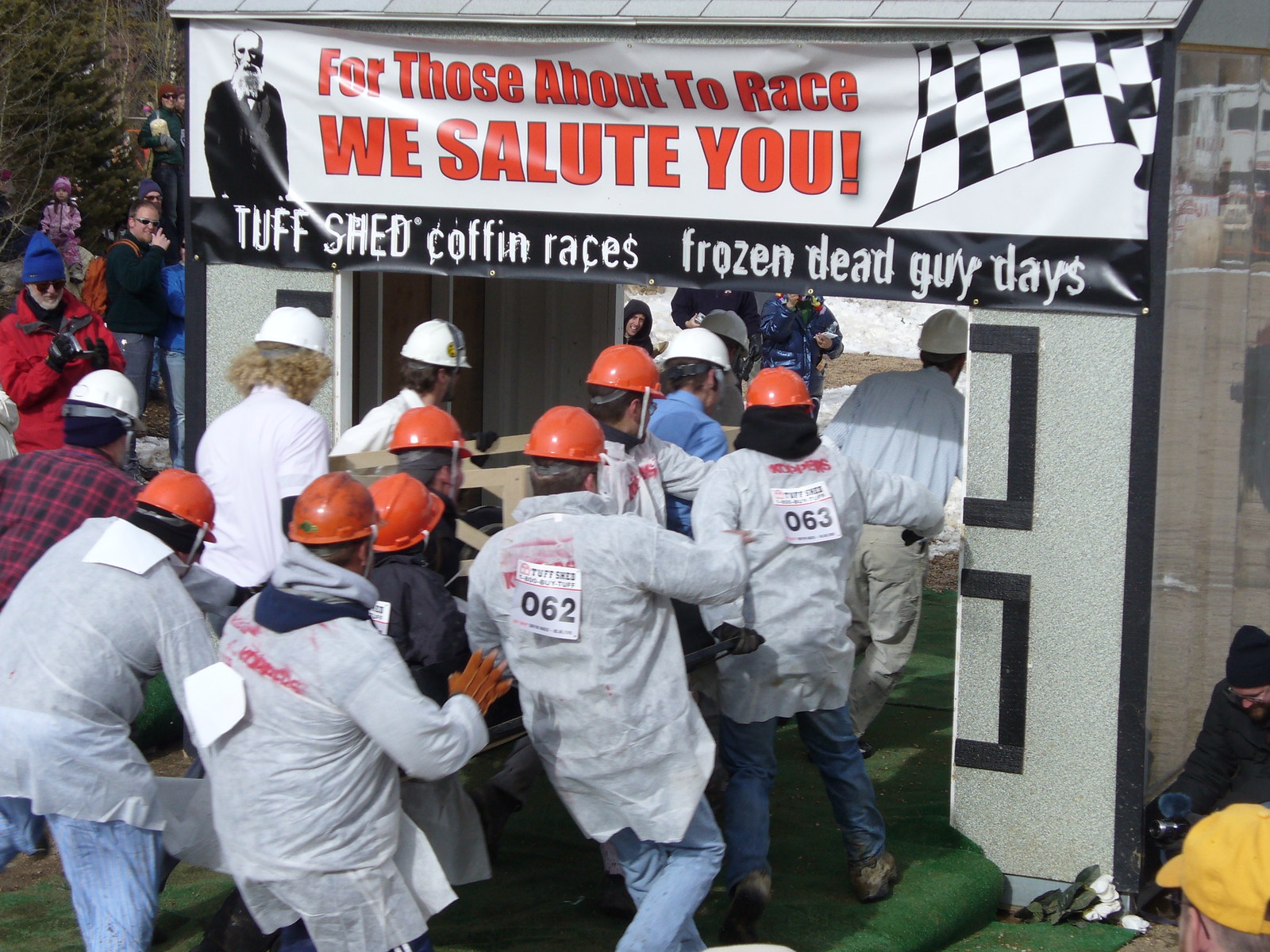The photograph captures a lively outdoor scene of workers participating in an event, moving through a green-carpeted entryway beneath a large archway. The workers, mostly men, are uniformly dressed in protective white jackets and various colored hard hats—primarily orange with some white. Each jacket has a number taped to the back, such as 062 and 063. Above the archway, an eye-catching white banner with bright orange text reads, "For those about to race, we salute you," accompanied by a checkered racing flag and an image of an old man with a beard. Below this, a black banner states, "Tuff Shed Coffin Races, Frozen Dead Guy Days." In the foreground, several workers with orange helmets and white overcoats can be seen, while in the background, more participants in white hard hats also prepare to enter. Onlookers are gathered on either side of the archway, adding to the sense of anticipation and excitement.